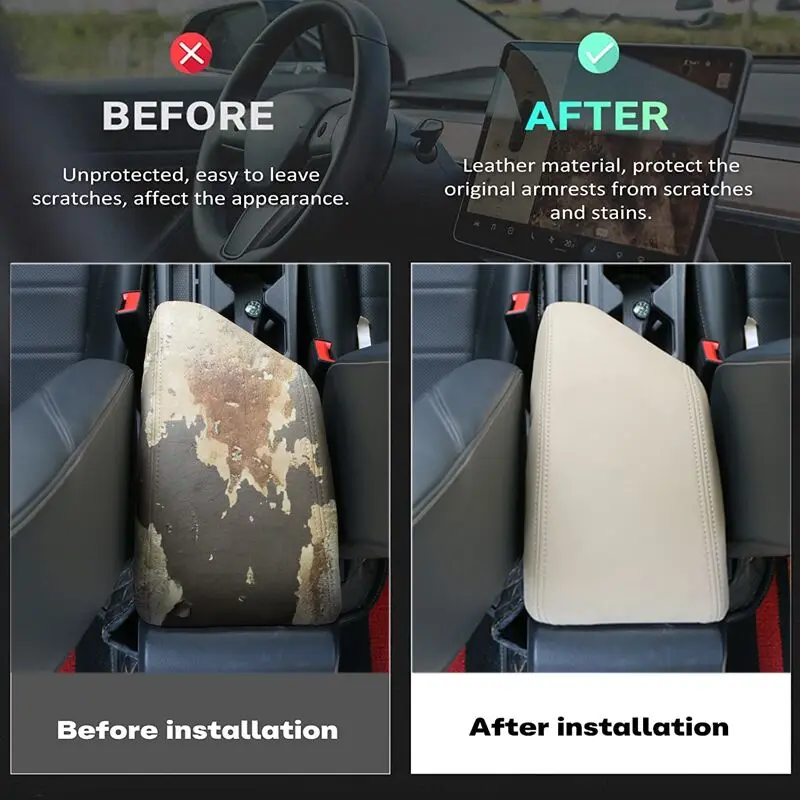This advertisement poster vividly illustrates a before-and-after demonstration of a car's center console upholstery enhancement. In the "Before" section on the left, marked with a big red X and captioned "unprotected, easy to leave scratches, affect the appearance", the bird's-eye view reveals a severely worn-out center console with visible scratches and stains. The accompanying text emphasizes the lack of protection leading to an unattractive interior. In contrast, the "After" section on the right, distinguished with a green check mark, showcases the same console now covered with a new, pristine leather material. The text here reads "leather material, protects the original armrest from scratches and stains," highlighting the product's effectiveness in safeguarding the console from future damage. This detailed demonstration features the color scheme of blue seats, a black steering wheel, and a black seatbelt with a red button, reinforcing the visual impact of the transformation. Overall, the advertisement underscores the product's capability to rejuvenate and protect car interiors from wear and tear.